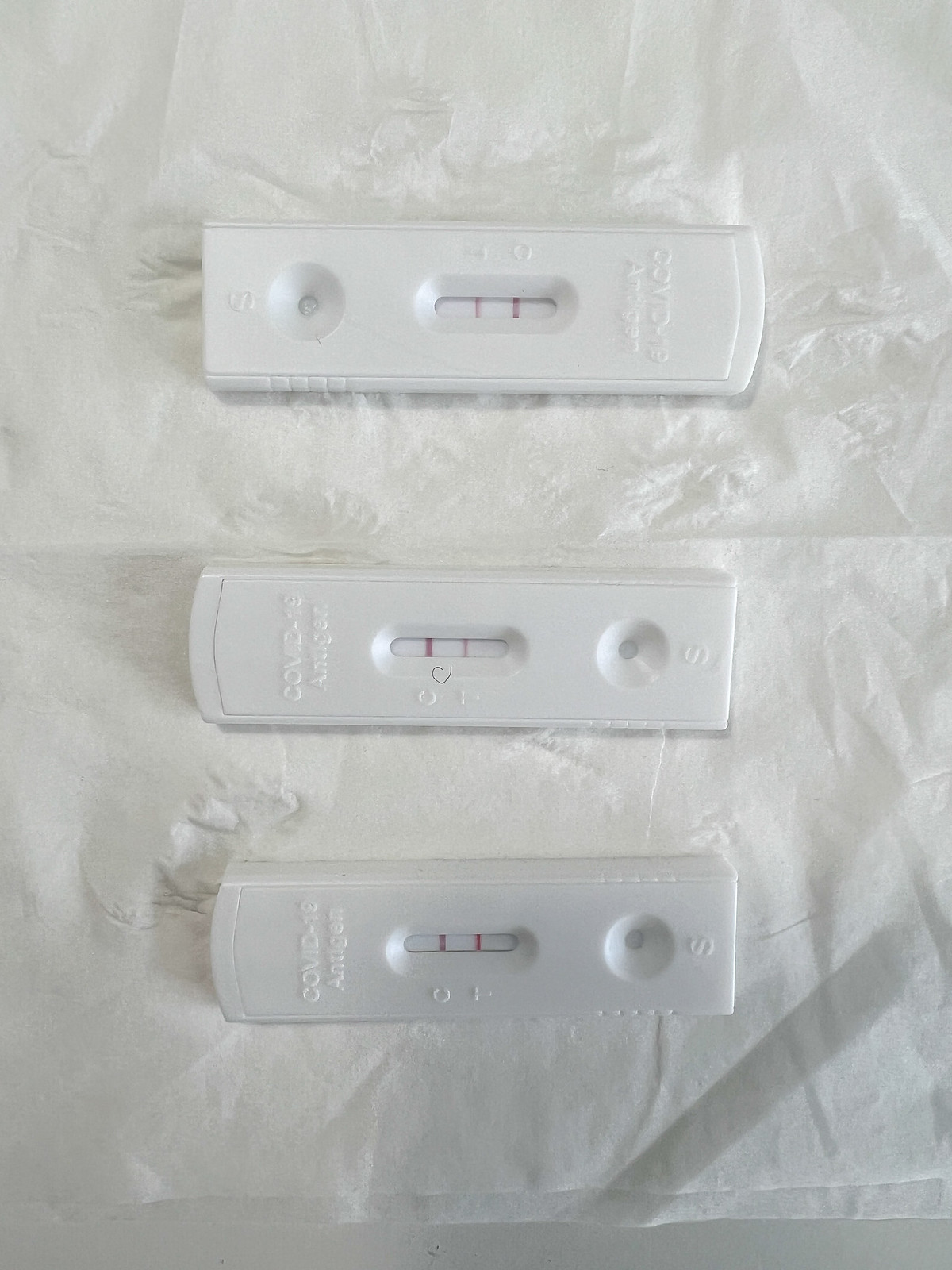The image features a close-up of three COVID-19 antigen tests placed horizontally on a crumpled white tissue background. Each test kit is made of white plastic and displays its results via colored lines next to labeled indicators. To read the text and interpret the results accurately, one must turn their head to the right.

The test at the top has "COVID-19 Antigen" labeled prominently. The left side shows a red line marked "C" for control, indicating the test is valid. Next to it, a faded green line marked "T" suggests a positive result. Below these indicators is a circle labeled "S," likely where sample drops were added.

The middle test, oriented opposite to the top one, requires tilting your head to the left. A faint piece of hair or dirt is visible near the "C" control line, which is dark red, signifying a positive result. The "T" test line is also marked, confirming the positive indication.

The bottom test is similarly oriented as the top one and also shows a positive result, with both the "C" control and "T" test lines clearly marked.